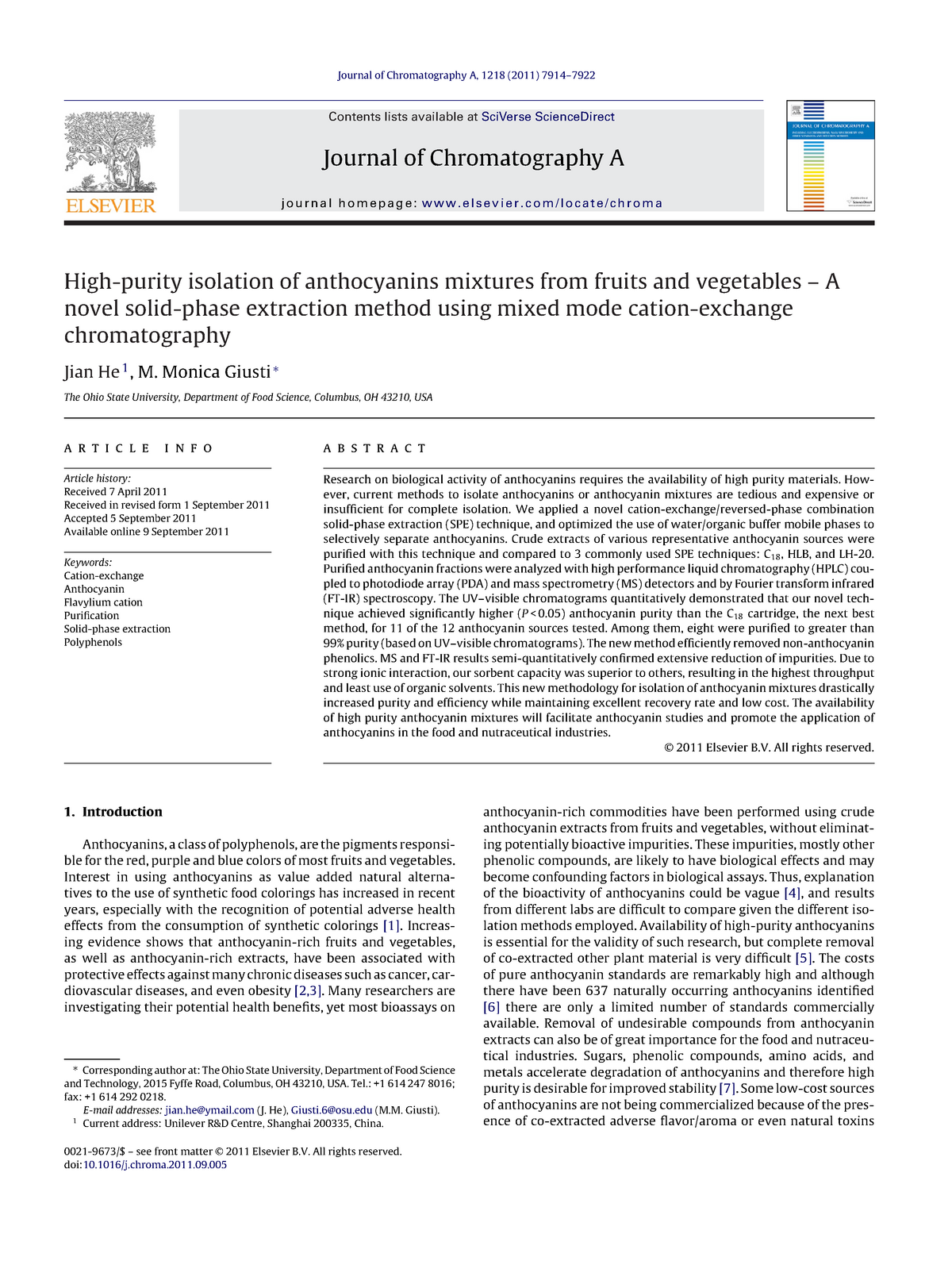The image depicts a page from the "Journal of Chromatography A", a scientific publication focused on chromatography. The top section of the page features a white background with blue text, prominently displaying the journal’s name— Journal of Chromatography, A— along with additional numerical identifiers indicating the volume and issue numbers, which help locate this specific page within the journal.

At the top of the page, a bar is divided into sections: the leftmost section bears the Elsevier logo, the publisher of the journal. The logo consists of a stylized image depicting a person beneath a tree, accompanied by the publisher's name, Elsevier.

Beneath this top bar lies the title of the featured article: "High-Purity Oscillation of Anthocyanin Mixtures from Fruits and Vegetables: A Novel Solid-State Phase Extraction Method Using Mixed-Mode Cation-Exchange Chromatography." This is followed by the authors' names, and their affiliations highlighted as the Ohio State University, Department of Food Science, Columbus, Ohio, including the relevant zip code.

Following the title and author information is a section titled "Article Info," occupying about a third of the horizontal space. This section provides additional details such as submission dates, acceptance dates, and other bibliographic information. Adjacent to this, on the right side, is the abstract of the article, summarizing the key findings and methodologies used in the study.

The lower section of the page transitions into the main body of the article, beginning with the introduction. The content appears to be scrollable, allowing readers to navigate through the entire article for an in-depth review.